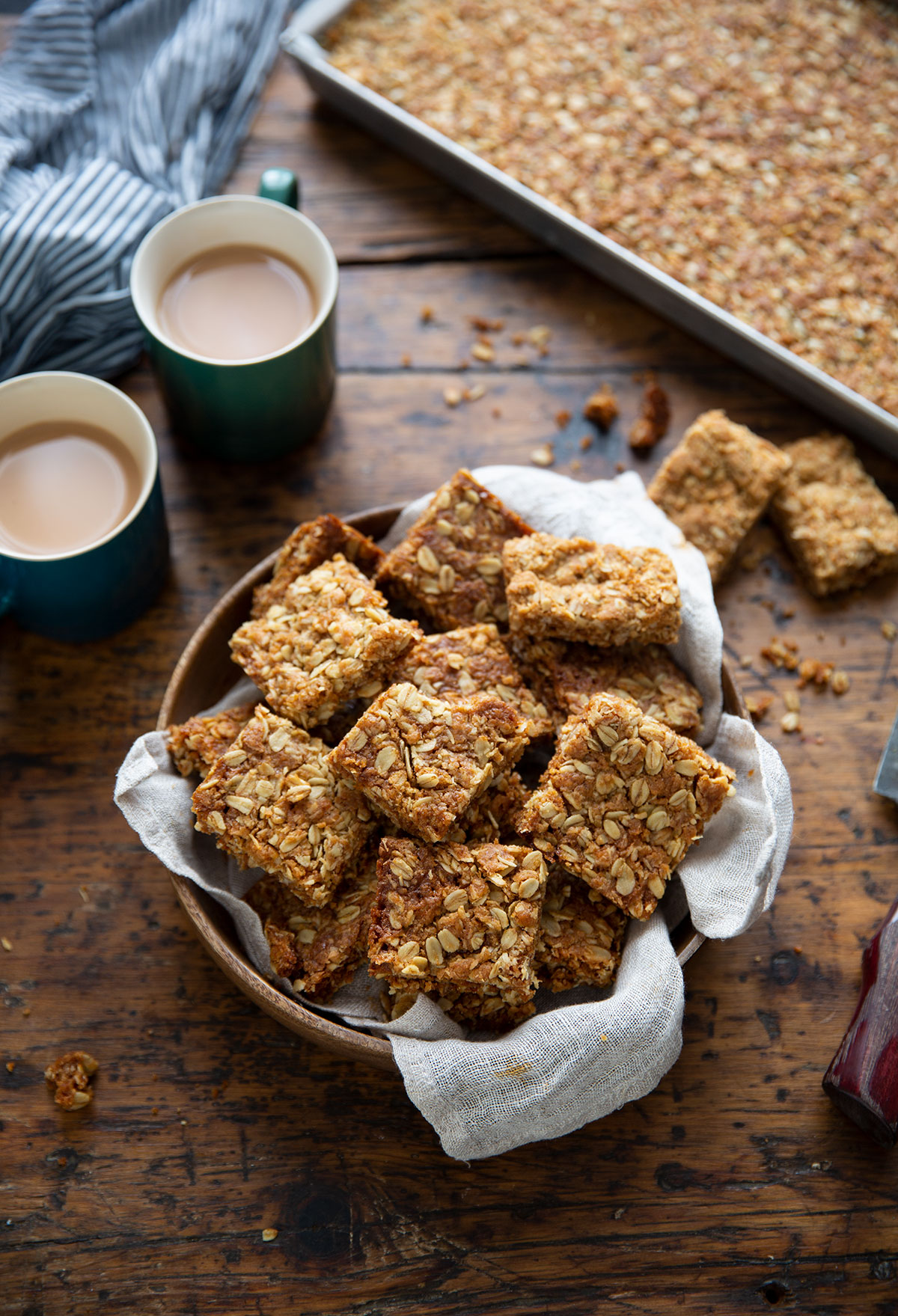This detailed top-down image captures a rustic scene centered around a wooden bowl lined with white cheesecloth, containing several homemade oat bars segmented into squares. The golden-brown treats are sprinkled with oats and present a freshly baked appearance. Surrounding the bowl, particularly to its right, are a few scattered oat squares with crumbs suggesting their recent relocation. In the upper right corner, a metal baking pan holds the uncut remainder of the batch. On the aged, dark-knotty wooden table, which adds a touch of character with its perceived wear and tear, two coffee cups with light-colored coffee sit snugly together in the top left region of the image; one cup is blue, and the other is green. An adjacent blue and white striped apron completes the cozy, homemade ambiance.